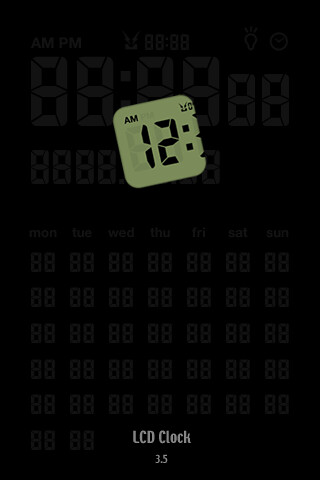A digital LCD clock with a brownish-gray display is showcased in the image. On the left side of the screen, the label "AM" is visible. The time display prominently features the digits "12" in the middle, followed by a colon and additional digits. A black mark is noticeable in the top right corner of the display. The background reveals faint, grayed-out segments that could be illuminated to form other numbers or indicators such as "PM."

The upper portion of the display contains large, segmented patterns that resemble the number 8, designed to form various digits when activated. The central section displays the sequence "8 8 8 8," indicative of its digital format. At the bottom, day abbreviations are listed: "MON, TUE, WED, THU, FRI, SAT, SUN," each separated by spaces. Beneath these day indicators are vertical columns of unlit segments showing "8 8."

The red box surrounding the display identifies the device as "LCD Clock 3.5."